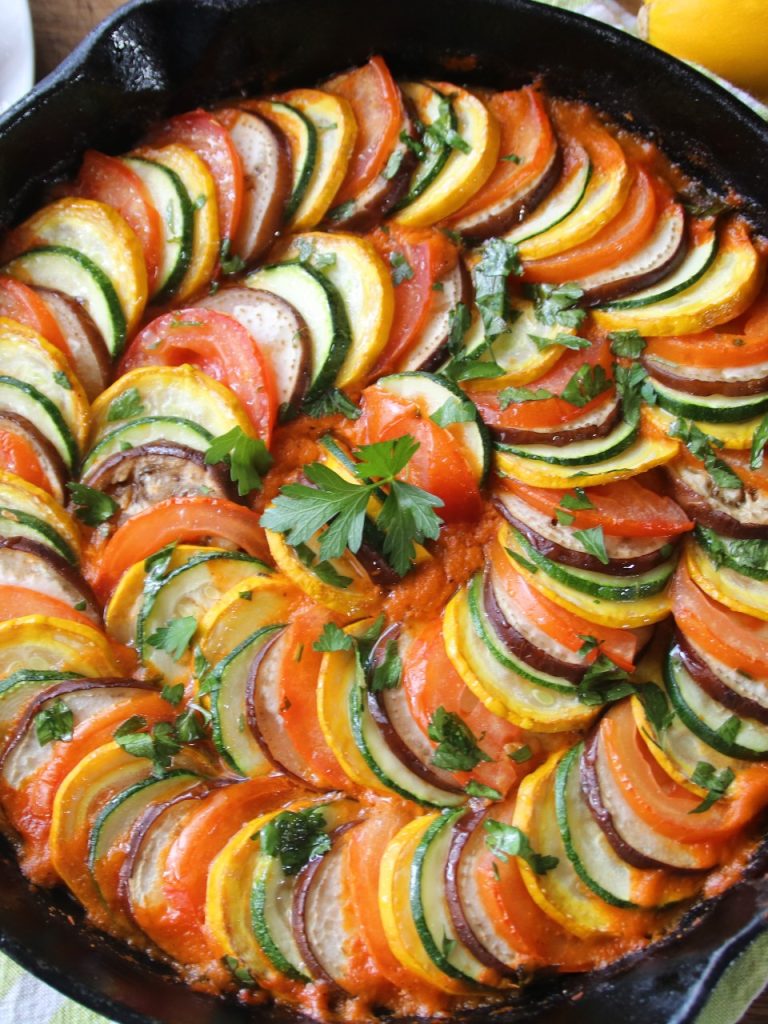The image depicts a beautifully arranged ratatouille in a large, shiny black skillet. You can see thinly sliced vegetables, including green zucchini, yellow squash, and red tomatoes, layered meticulously in a circular, spiral pattern. The vibrant vegetables are cut into precise, coin-like shapes, creating an eye-catching contrast of colors. Each slice is stacked neatly, forming a visually appealing design that fills the entire pan. Sprinkled on top, adding a touch of freshness, is green parsley. The base of the skillet is coated with a rich tomato sauce, which can be seen peeking through between the vegetable layers. In the background, a green and white tea towel is visible in the left-hand corner, along with the edge of a yellow vegetable on the right and a brown table surface in the left corner. This detailed arrangement showcases a classic ratatouille, both aesthetic and appetizing.